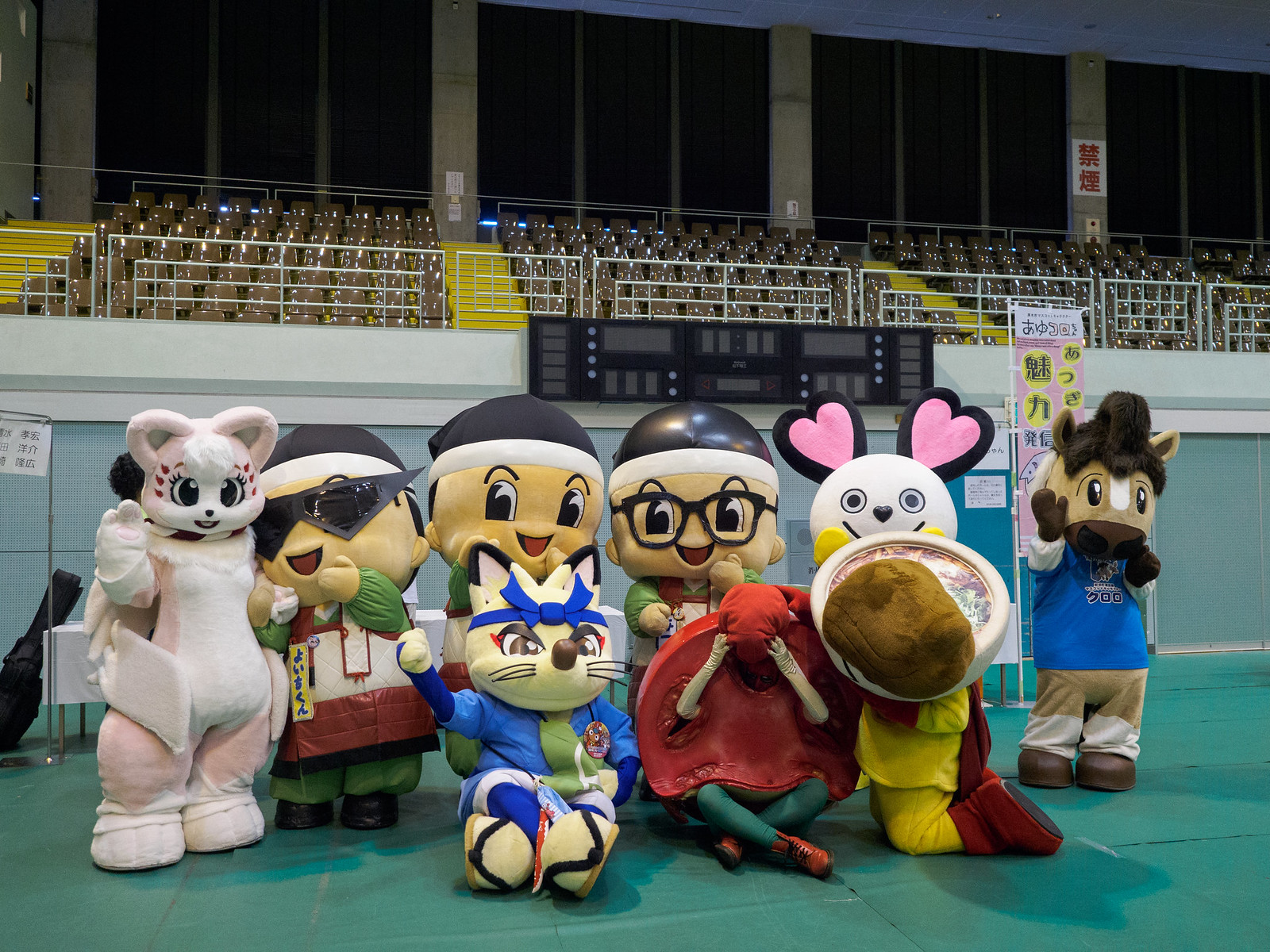In this vibrant and detailed photograph, we see nine cartoon-themed mascots set against the backdrop of a large, green-floored sports complex or auditorium, complete with rows of tiered bleacher seats and a blue wall. The mascots are arranged in two rows, with six standing in the back and three seated or kneeling in the front. Starting from the left, the lineup begins with a pink, female cat mascot, characterized by white trim, red whiskers, and a big smile. Next to the cat is a small child-like figure wearing triangle-shaped sunglasses, a red and white t-shirt, and an apron over green attire. This figure has an off-white tan face and black shoes.

The third and fourth mascots resemble the Mario Brothers, both donning black and white hats, and one of them is sporting glasses. An off-white kitten with a bright blue bowtie, brown eyes, and a blue shirt sits in front of the Mario-like characters, flaunting flip-flops with a crisscross pattern on the toes.

On the far right of the back row stands a white-headed mascot with pink heart-shaped ears, adorned in what appears to be a yellow outfit. Moving further right, a tan-furred mascot with a brown hat, black eyes, and beige pants is waving, dressed in a blue shirt and brown shoes.

In the front row, aside from the aforementioned kitten, there is a round, unidentifiable mascot with green legs, red shoes, and beige gloves – possibly representing a sliced tomato. The final mascot seated in the front features tan fur and traditional Japanese garb, enhancing the diverse assembly of characters. This captivating arrangement provides a feast of colors and shapes, set against a seemingly empty venue, offering a whimsical yet orderly portrayal of these playful figures.